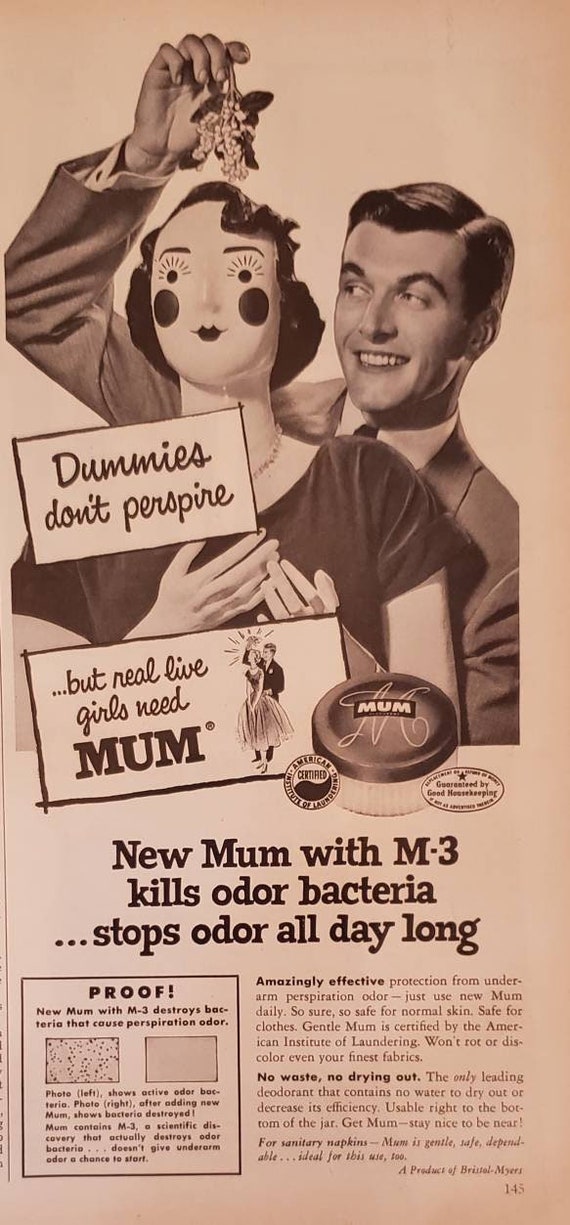The image is a vintage advertisement featuring a Caucasian man dressed in a suit, white shirt, and tie, standing behind a woman who appears to be a dummy or puppet. The dummy woman, also Caucasian, has black hair, wears a black dress with a necklace, and has a head resembling a mannequin with face paint and a wig. The ad, set against a light peach background, promotes an old-fashioned deodorant called "mum". The text on the image reads, "Dummies don't perspire, but real life girls need mum," indicating the product's promise to control underarm odor. There is a small canister of the product labeled "new mum with M-3" which claims to "kill odor bacteria and stop odor all day long". Additional text mentions the product is "amazingly effective," with endorsements from Good Housekeeping, its safety for normal skin and clothes, and the importance of daily use for optimal results. The advertisement appears to be a reproduction from a magazine or newspaper, possibly with fine print detailing further product benefits.